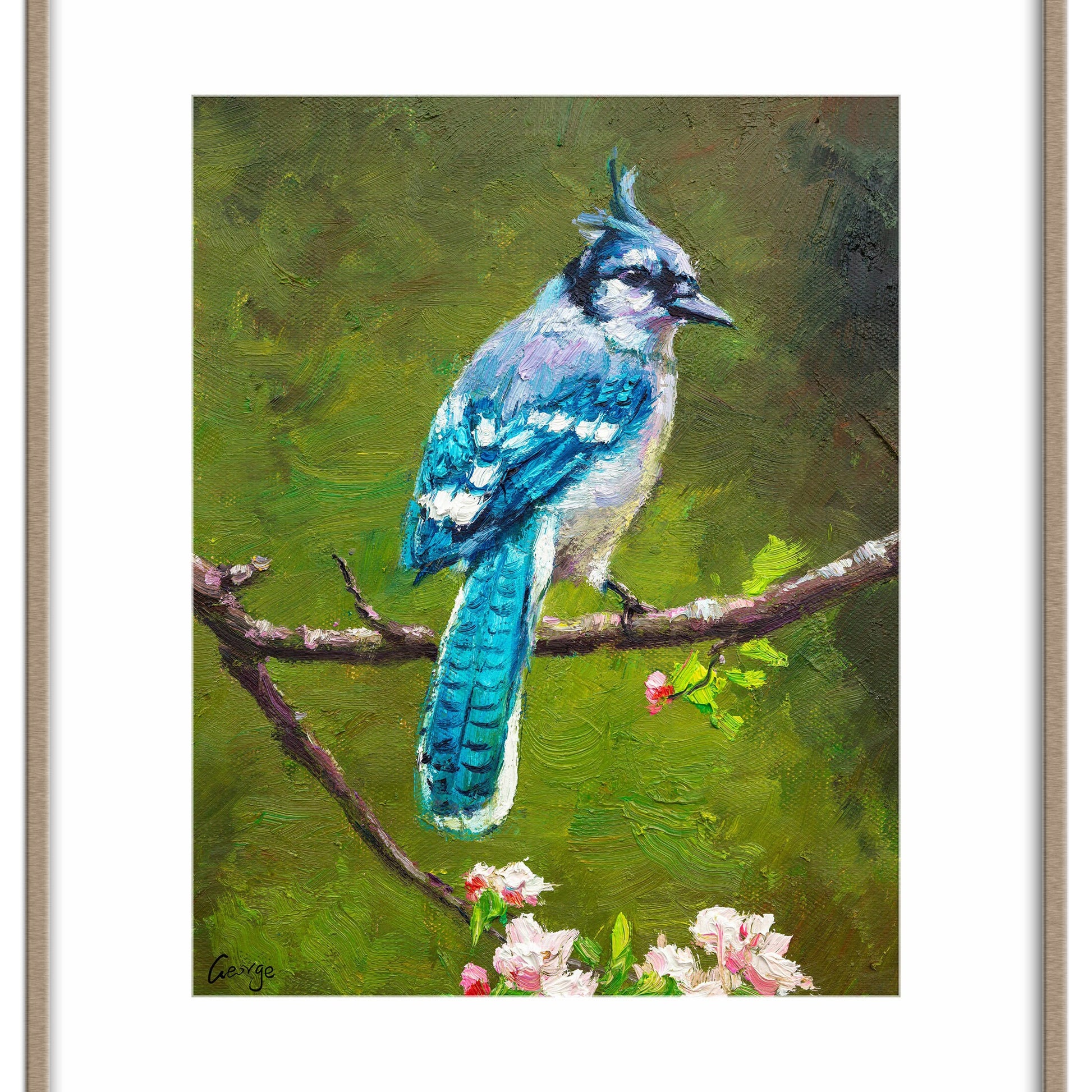In this detailed painting, set against a white background, we observe a vibrant blue jay perched on a brown branch, interconnected with another that bears blooming flowers. The background is a lush green with hints of nature. The blue jay, primarily light blue, features distinctive spiky teal feathers atop its head and white surrounding its eyes. Its head, sporting a grayish-blue beak, is turned back towards us while its body faces away, slightly to the right. The bird’s wings showcase a mix of blue with white spots, and its tail feathers are vividly teal and white. Notably, the bird's legs are black and its neck area has a touch of black. The branch it rests on extends horizontally, adorned with pink and white flowers and green leaves on the right side. Additionally, a smaller branch descends with clusters of petals blooming around it, enhancing the picturesque scene.